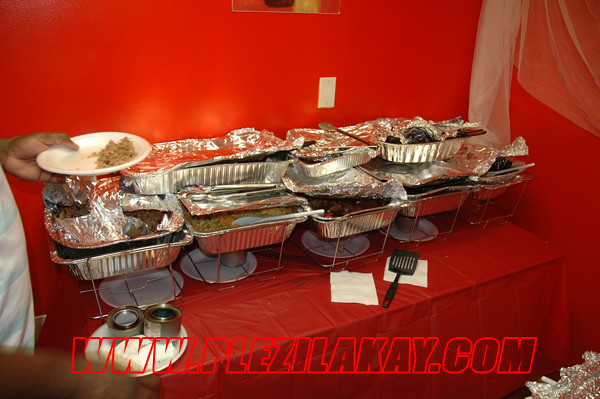In this vibrant color photograph, a festive buffet setup is displayed inside a red-walled tent. The serving table, covered with a reflective red waterproof tablecloth, supports a bountiful spread housed in large aluminum trays, some of which are sealed with aluminum foil while others are accessible with tongs for serving. The trays are arranged on metal racks designed to keep the food warm. Positioned directly above the table is an electric plug-in. 

On the table, towards the front, lie two napkins with a black spatula resting on the one to the right. Plates are visibly stacked behind the napkins and underneath the trays. To the left of the frame, a gentleman partially enters the shot, identifiable by his chest, left hand, and white plastic plate, which holds a serving of rice and is marked with the text "www.poliske.com." The scene suggests a catered event with consistent red decor, possibly reflecting a wedding theme, underscored by a white fabric element reminiscent of a bridal veil draped against the red walls. 

Text reading "www.plezilakay.com" is noticeable at the bottom of the image, matching the red color scheme. Additional details include the outline of a hand blurred at the bottom left and a crystal-like gray object in the bottom right corner of the frame, enriching the overall visual narrative.